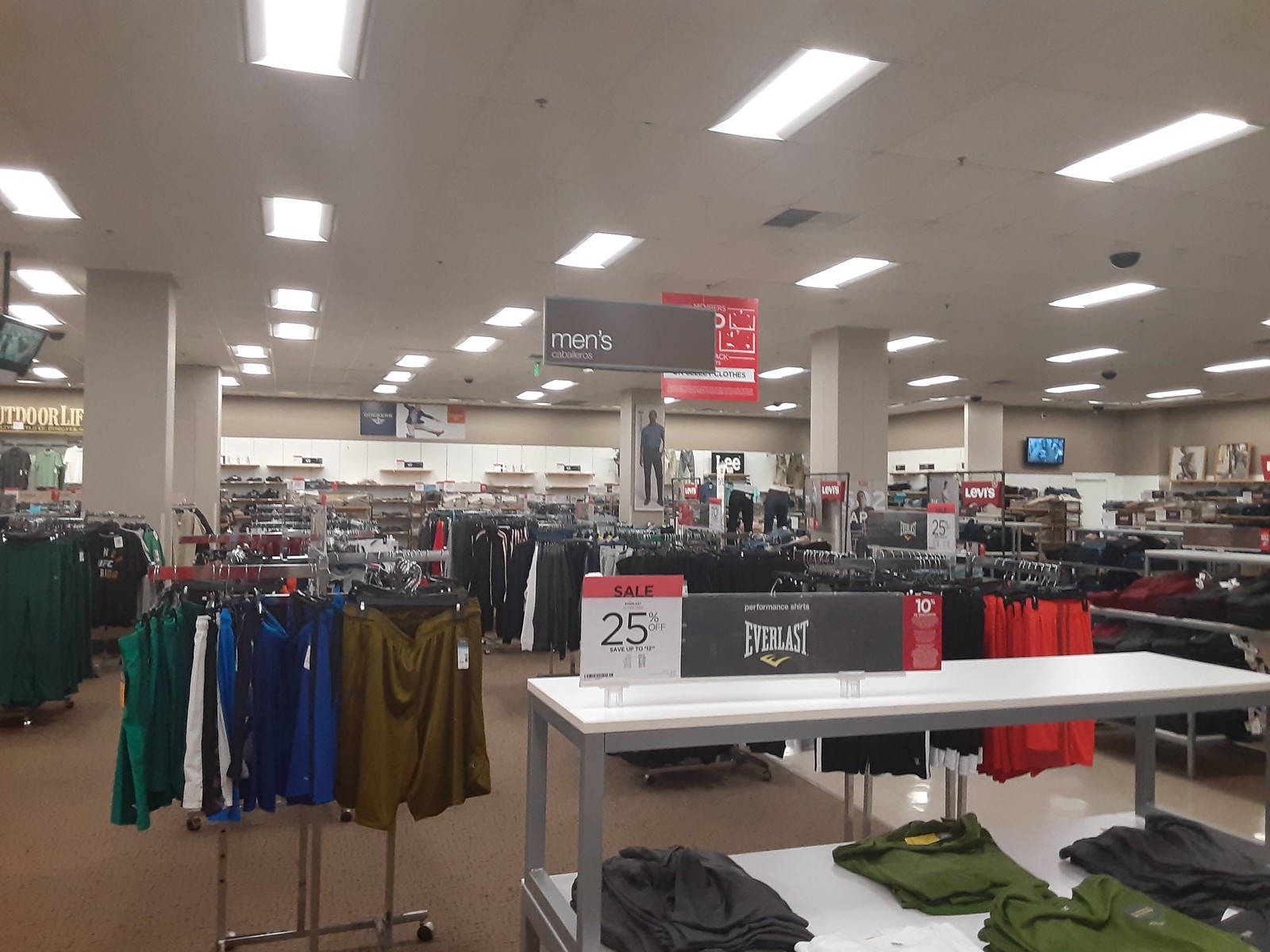This detailed caption for the photograph of a large indoor clothing store should encapsulate its essential features:

---

The photograph captures the expansive interior of a large clothing store, showcasing its bright, white ceiling adorned with large rectangular strobe-style lighting fixtures. The store is organized with racks situated in the middle, primarily displaying men's shorts and trousers, accompanied by a prominent overhead sign indicating the men's section. A nearby shelf brims with meticulously folded t-shirts, highlighted by a "Sale 25% Off" sign, inviting shoppers to peruse discounted items. The store offers a variety of different brands, and a substantial shoe display is visible at the back of the store. On the walls and suspended from the ceiling, multiple TV screens or CCTV monitors can be seen, adding to the modern retail environment. The layout and product offerings suggest the store specializes in outdoor clothing.